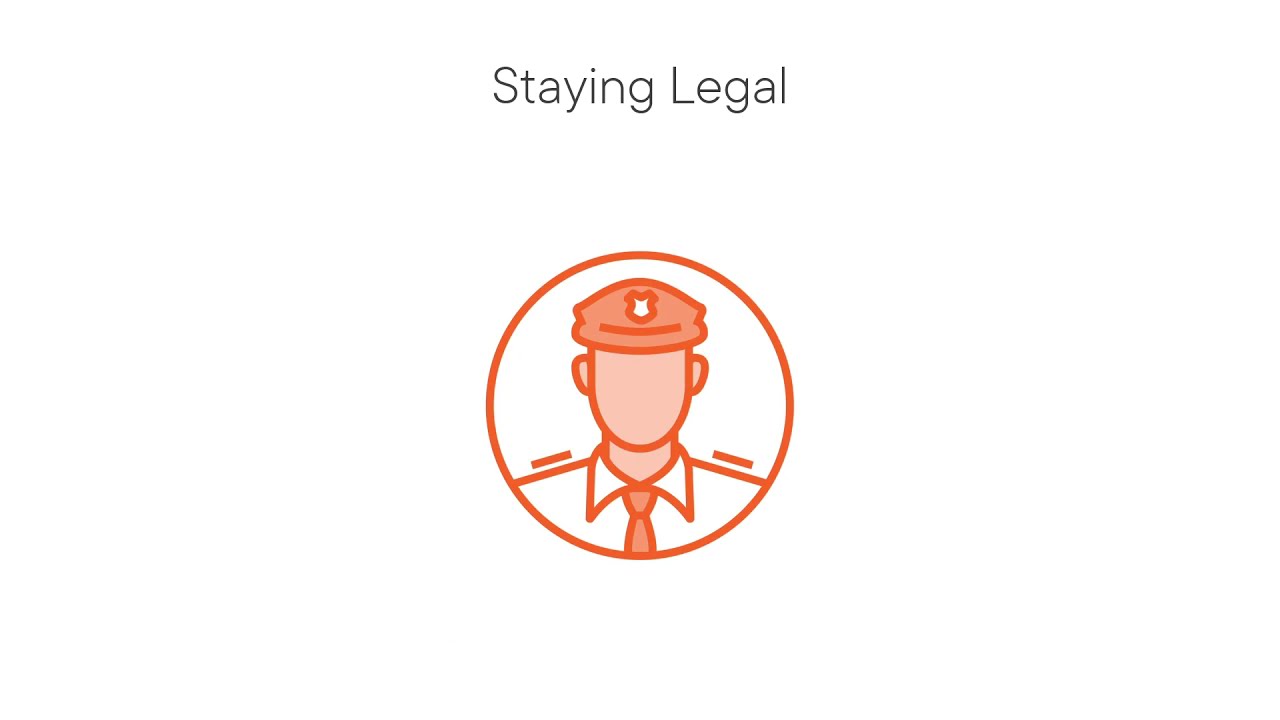The image is a minimalist design with a completely white background and black Arial font at the top saying "Staying Legal," with the 'S' and 'L' capitalized. Below this text, there's an orange circle containing a simplified, faceless outline of a police officer or military figure. The figure is rendered in shades of orange and white, wearing an orange hat with a white badge emblem and a white collared long-sleeved shirt with an orange necktie that has darker orange trim. His shoulders are accented by two small parallel orange lines, suggesting insignia or badges. The overall aesthetic is clean and modern, emphasizing the themes of legality and authority through its stark, straightforward imagery.